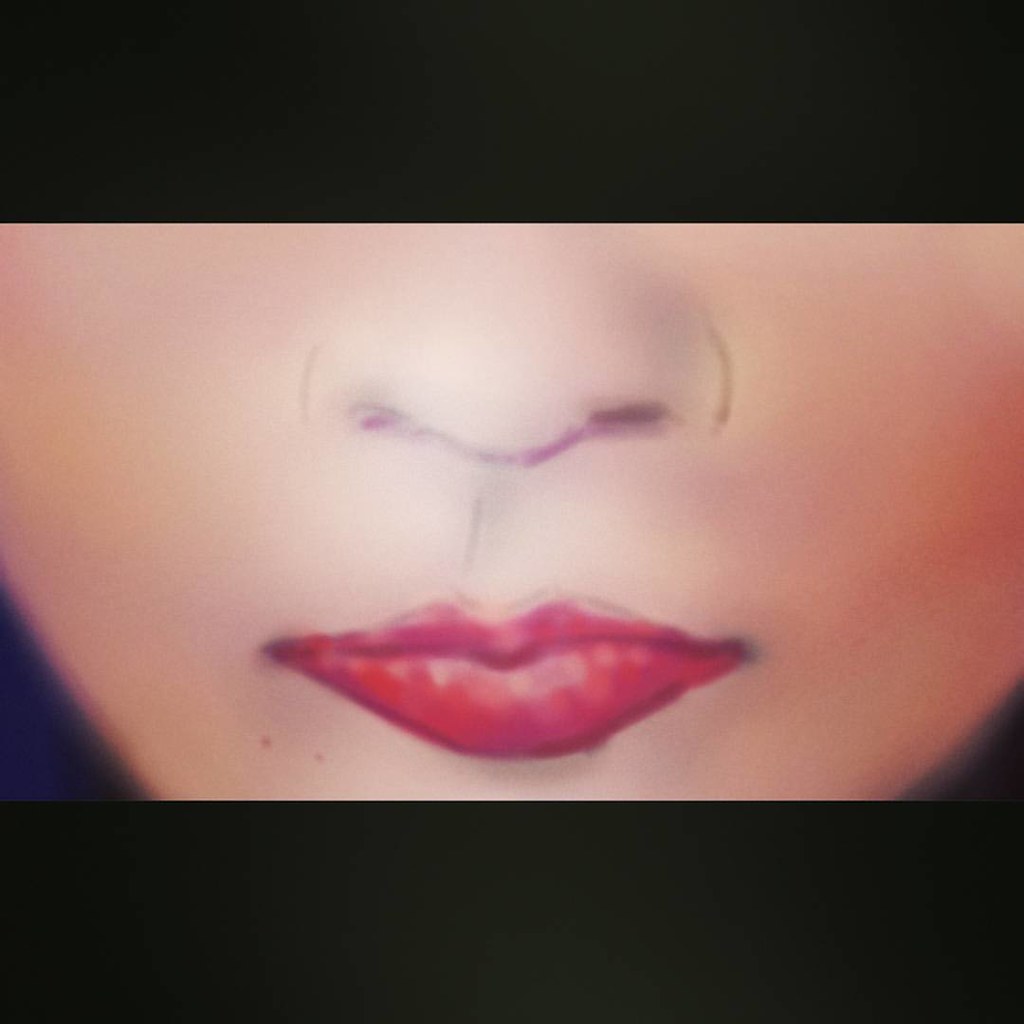The image is a slightly taller-than-wide, letterboxed painting or cartoon that captures the lower two-thirds of a young Caucasian woman's face. Dominated by a black horizontal band at the top and bottom, the central area features a detailed, zoomed-in view of her facial features from just above the nose down to the chin. Her skin is light, and she wears vibrant red lipstick that is neatly outlined. The nose is subtly sketched with just the nostrils and the two curves marking its sides, lacking a detailed bridge. The jawline is V-shaped and the background around her face is black, adding contrast to the central image. The overall look suggests a hand-drawn or painted style, though it has a clean, possibly airbrushed or computer-animated feel.